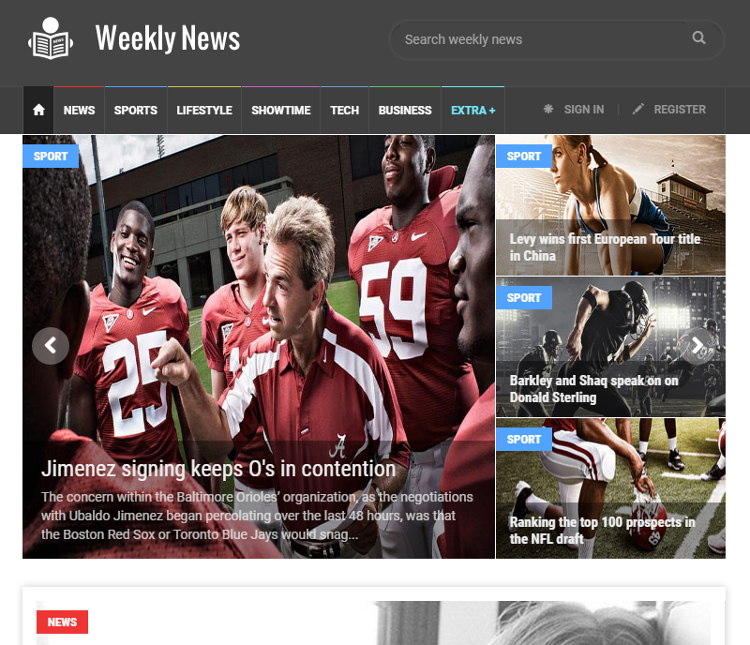Homepage of Weekly News: Across the top is a charcoal gray banner running from left to right, adorned with crisp white text. On the upper left corner, an icon of a person reading a newspaper is prominently displayed, signifying the publication's dedication to delivering news. Adjacent to this icon, the text reads "Weekly News" in bold white letters. On the far right of the banner, an oblong oval with the words "Search Weekly News" followed by a magnifying glass icon invites readers to explore the site.

Directly beneath the banner, from left to right, small icons and text offer navigation options: a house icon representing the homepage, followed by white text labels for various sections such as News, Sports, Lifestyle, Showtime, Tech, and Business. Distinctly in blue text, "Extra Plus" stands out, alongside links for "Sign In" and "Register."

Dominating the center of the homepage is a large, vibrant image capturing the scene of a football team huddled around their coach. The players, clad in red and white uniforms, appear focused and engaged, embodying the intensity of the sport. There are approximately five players and one coach in this dynamic scene.

To the far right, three images are vertically stacked, each under the category "Sport" displayed in a blue rectangle on the upper left corner of each image. The top image features a Caucasian female celebrating her win, captioned "Levy wins first European Tour title in China." Below, an image of two football players in action accompanies the headline "Barkley and Shaq speak up on Donald Sterling." The bottom image showcases another football player in a crouched position, with the caption "Ranking the top 100 prospects in the NFL Draft."

This meticulously arranged homepage provides a comprehensive and engaging overview of the latest highlights and headlines in sports, seamlessly guiding readers through categories and notable stories.